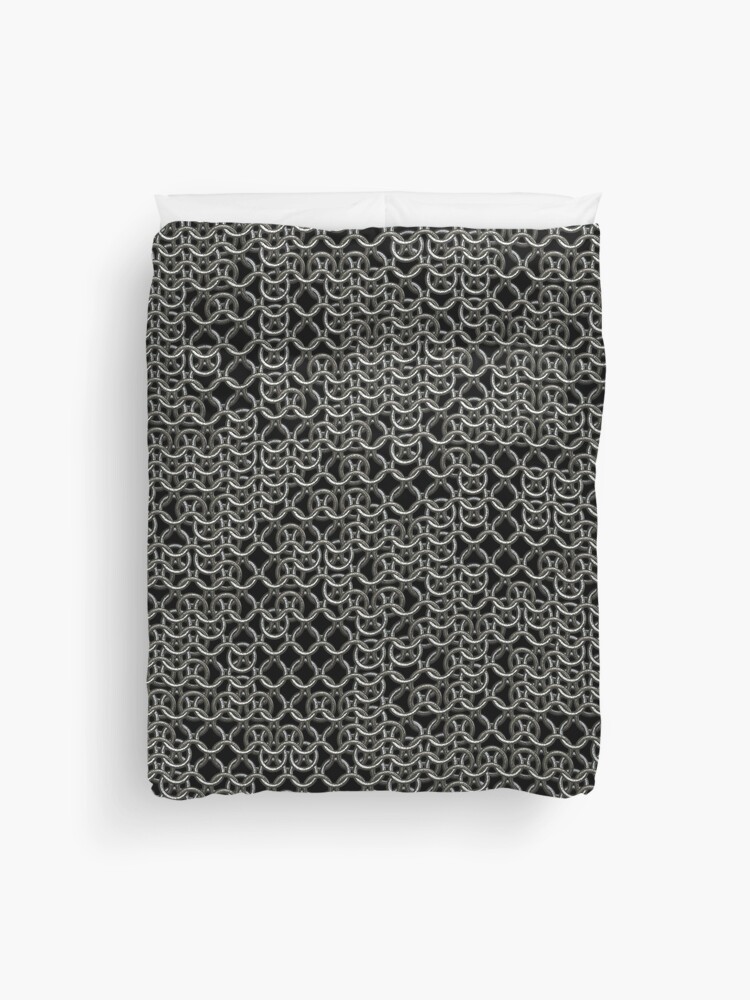The photo is of a bed with a white background and a white surface. On the bed lies a black pillowcase with a chainmail print. The print features interconnected, silver-gray circular hoops arranged in rows, creating the illusion of actual chainmail. The design has both tighter and looser groupings of circles, allowing the black background to show through more in certain areas. At the top of the pillow, about two inches of the white pillow inside is exposed, indicating that the pillowcase covers most of the pillow. The image captures a rectangular, vertically-oriented linen piece, possibly another pillow or a blanket with a chainmail pattern, further emphasizing the medieval chainmail texture. One can also observe a clear plastic bag near the top section, adding a realistic touch to the setting.